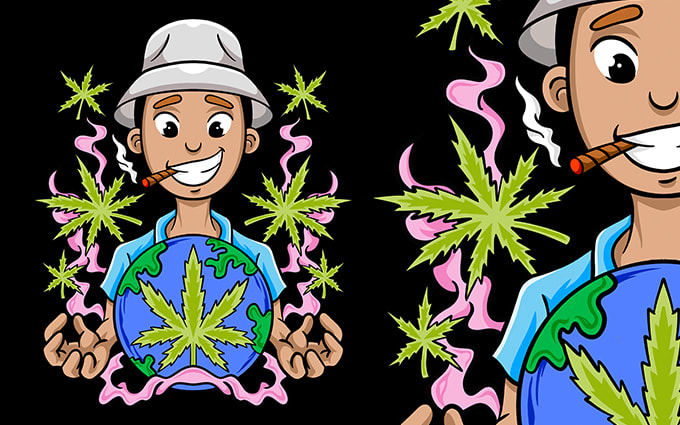This digital artwork features a cartoon character named Mal, who is depicted in a vibrant and engaging style. The image is split into two halves; on the left half, the full illustration is visible, while the right half showcases a zoomed-in version, displaying only part of the image. Mal is adorned in a white bucket hat and a blue shirt, with a roll-up cigarette or joint in his mouth, emitting pink smoke that floats around him. He has a distinct smile on his face. In front of him, floating between his hands is a globe, prominently featuring a green cannabis leaf. Surrounding Mal's head are additional cannabis leaves, all set against a stark black background. The zoomed-in right side of the image highlights half of Mal's face, part of the globe with the cannabis leaf, and the surrounding pink smoke and marijuana leaves, creating a dynamic and captivating composition.